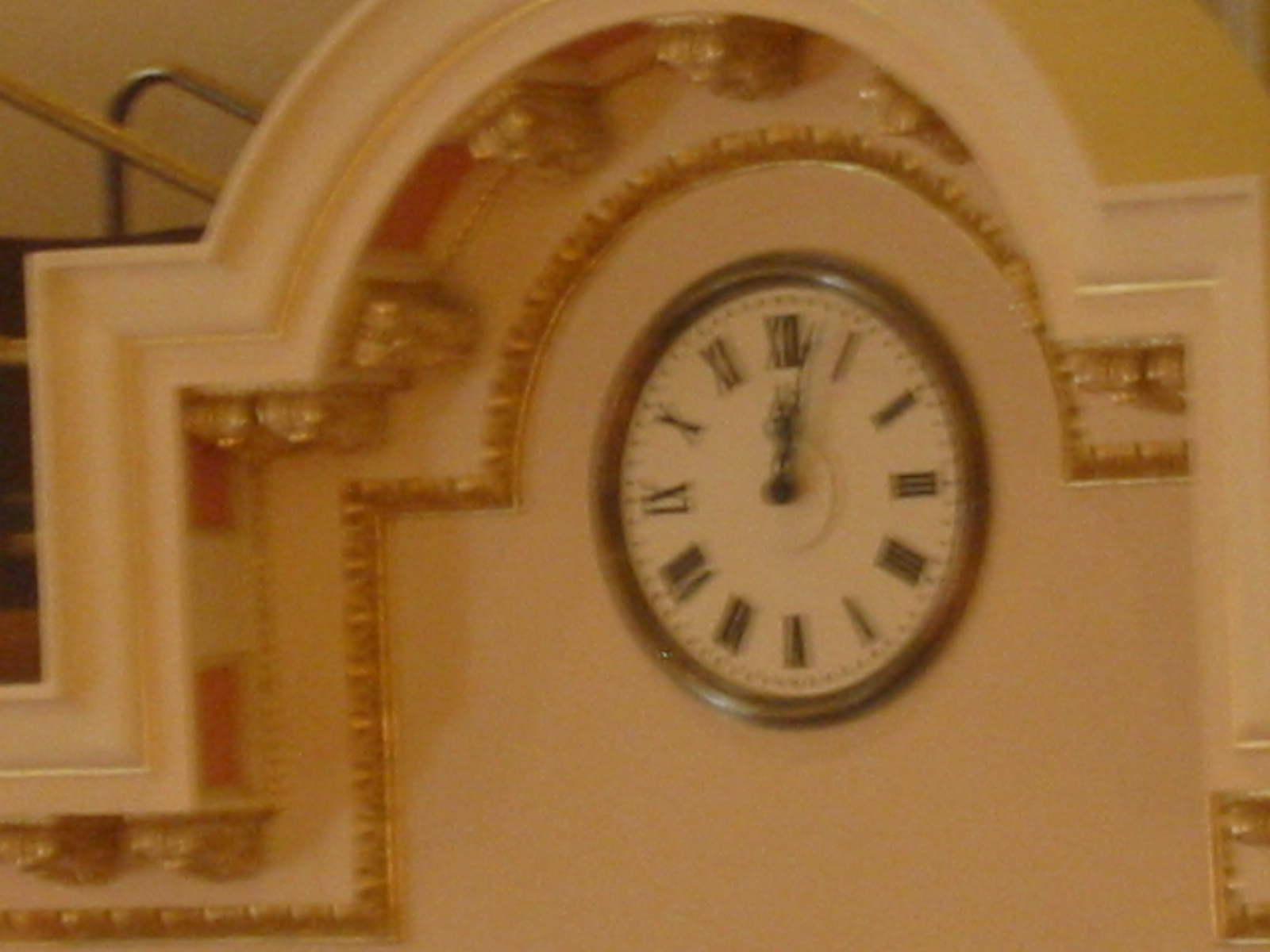This photograph captures a wall clock suspended within an elegant city building. The clock is mounted on an off-white wall adorned with a gold-painted, ornate design, beautifully complementing the arched section of the architecture. In the back left corner of the image, a staircase subtly reveals itself behind the wall, adding depth to the scene. The clock features a round frame in a brown or bronze hue, housing an off-white clock face marked with Roman numerals. The bronze or brown hands indicate the time as 12:02. Despite the slight blur, the image conveys a sense of classic charm, accentuated by the shadows on the left side and a glimpse of a yellow-painted wall emerging from the upper right of the arch.